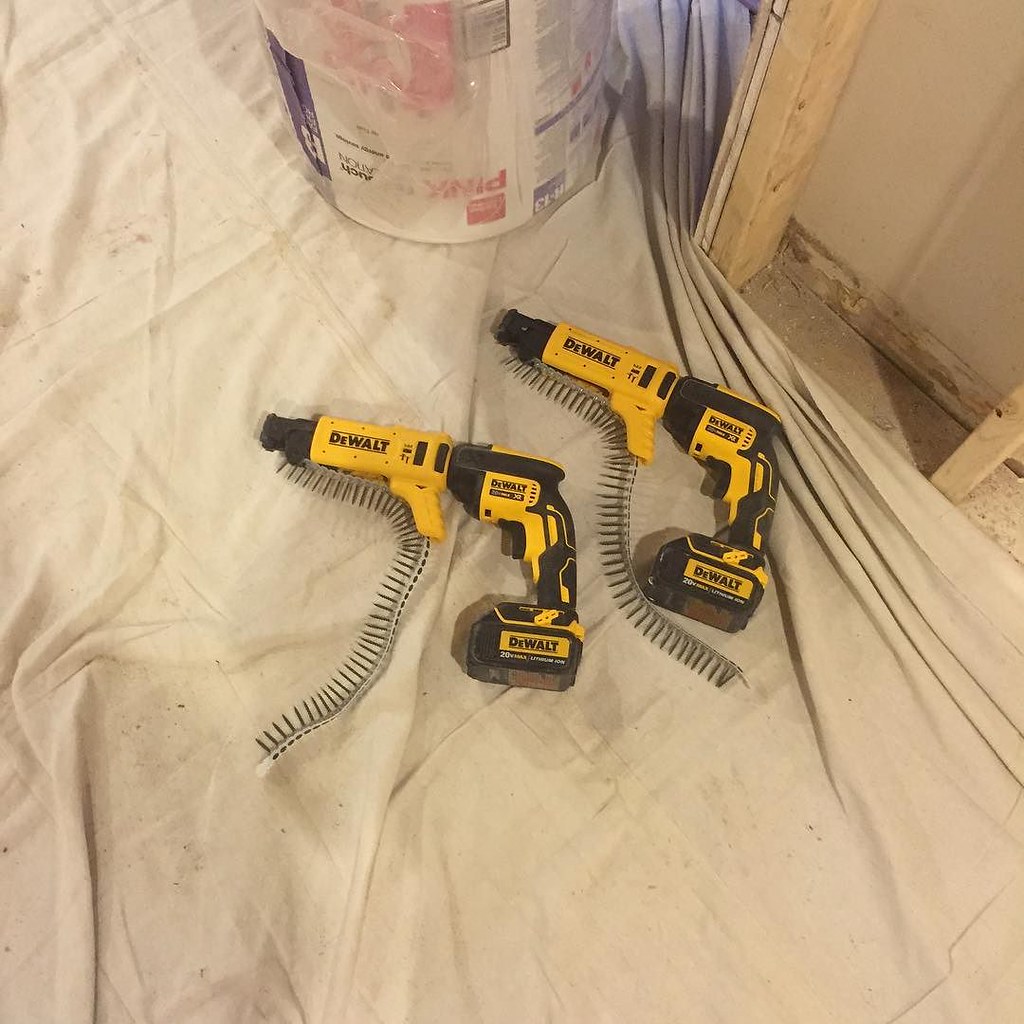The image is a color photograph depicting a home renovation or construction scene viewed from a high angle. The floor is covered with a slightly dirty, off-white light beige dust sheet, which is gathered and wrinkled towards the right side due to obstruction by a wooden post. Prominently placed on the sheet are two identical DeWalt nail guns, easily identifiable by their yellow and black bodies with the DeWalt branding. Each nail gun has a band of nails attached via a plastic strip, with the heads of the nails protruding through. In the top left-hand corner of the image, there is a blurred plastic bucket that appears to be holding some construction materials. The scene also shows the interior of a partially constructed wall in the upper right corner, featuring two spaced-out wooden struts with plasterboard set behind them. Dust and debris are visible on the exposed concrete floor around the perimeter of the dust sheet, reinforcing the ongoing nature of the renovation.